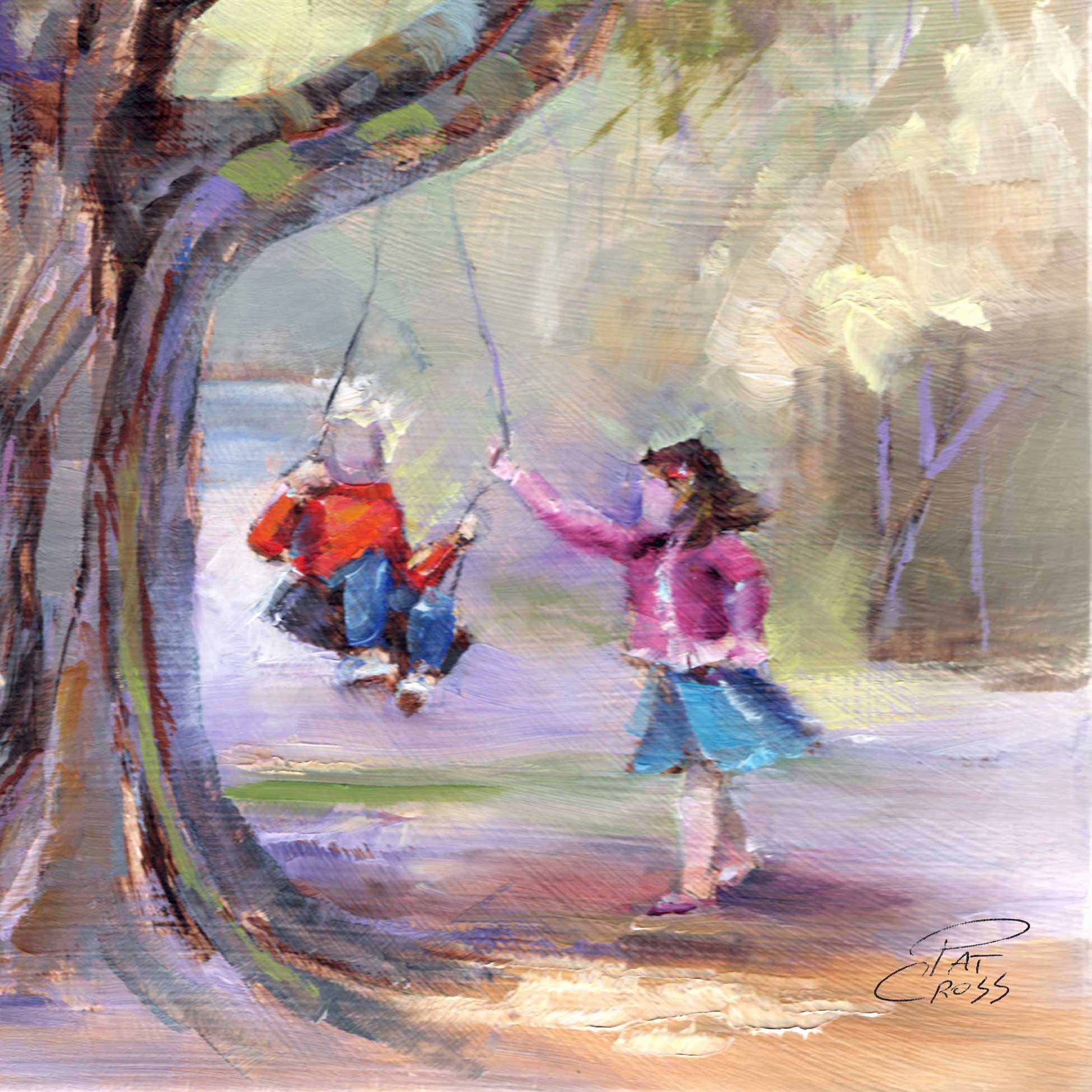The image is a watercolor painting by Pat Cross, signed in black at the bottom right corner. It has an abstract, blurry quality that leaves some details to the imagination. The scene, likely set in a park, features two children playing under a large tree on the left. The tree's trunk is brown with sprawling green leaves. A boy in a red shirt, blue jeans, white sneakers, and a gray hat is blissfully swinging on a swing with a black seat, holding onto the ropes. A girl, identified by her pink jacket and blue skirt, with dark brown hair, stands next to him, pulling the rope to give him momentum. The background is softened by sunlight, casting a warm glow and highlighting other trees with whitish beige leaves, giving the whole painting a serene, pastel vibe. The children’s faces are notably absent, adding to the abstract nature of the artwork.